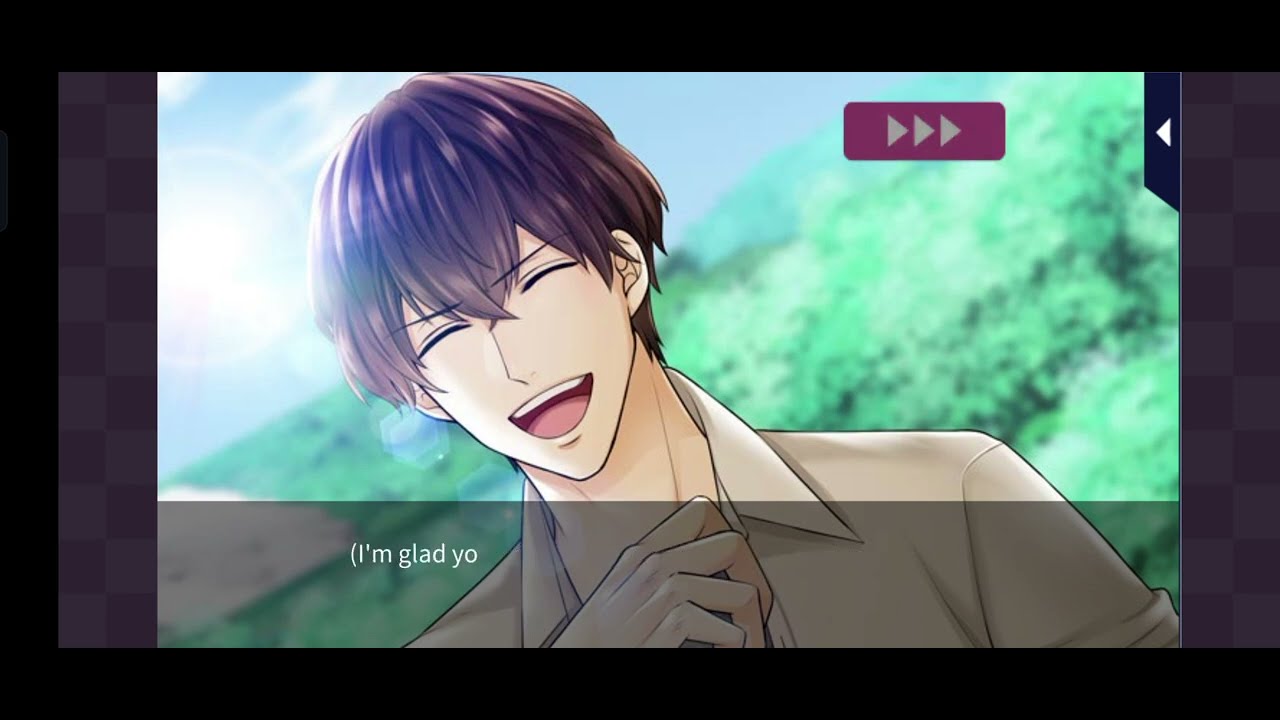The image is a detailed screen grab from an anime cartoon, framed by a thick black border. The central figure is a light-skinned, short brown-haired male character with his head tilted slightly to the left. His eyes are closed, his mouth is open in a laughing expression, and his right hand is raised to his neck level. He is wearing a tan collared shirt that appears open at the front. The background is a green, faded landscape with hints of sky at an angle. In the upper right corner of the image, there is a maroon rectangle with three white triangles pointing to the right. Additionally, a small black horizontal line with a white arrow points to the left. The bottom center of the image contains cut-off subtitles that read, "I'm glad yo."